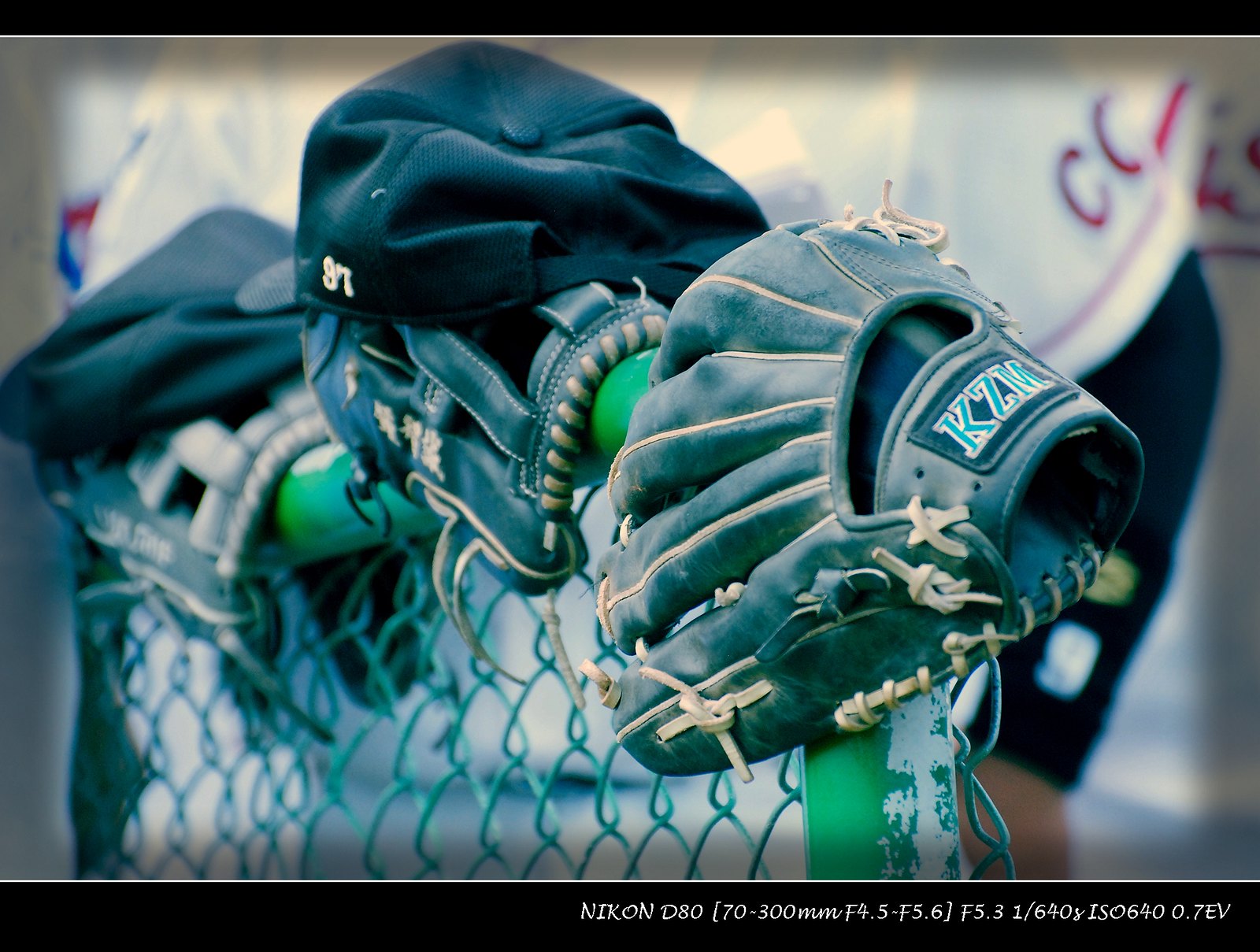The photograph depicts three baseball gloves carefully balanced on a green chain-link fence, with two of them adorned with baseball caps. The gloves and caps have a striking green color with white striping and letters, notably "KZM" visible on one glove. The first glove, positioned at the edge of the fence, stands out without any cap. The middle gloves each support a green baseball cap with the number "97" on it. The scene is set in a ballpark, and the fence shows signs of wear, with chipped paint revealing its age.

In the background, a baseball player in a white jersey with "CC" in red letters on the shoulder and a red stripe stands prominently. The player's dark long-sleeved shirt peeks out beneath the jersey. Towards the bottom of the image, in a black bar, the camera details are printed: "Nikon D80 70-300mm F/4.5-5.6 1/640 ISO 640". The overall color scheme and details suggest a nostalgic sports atmosphere.